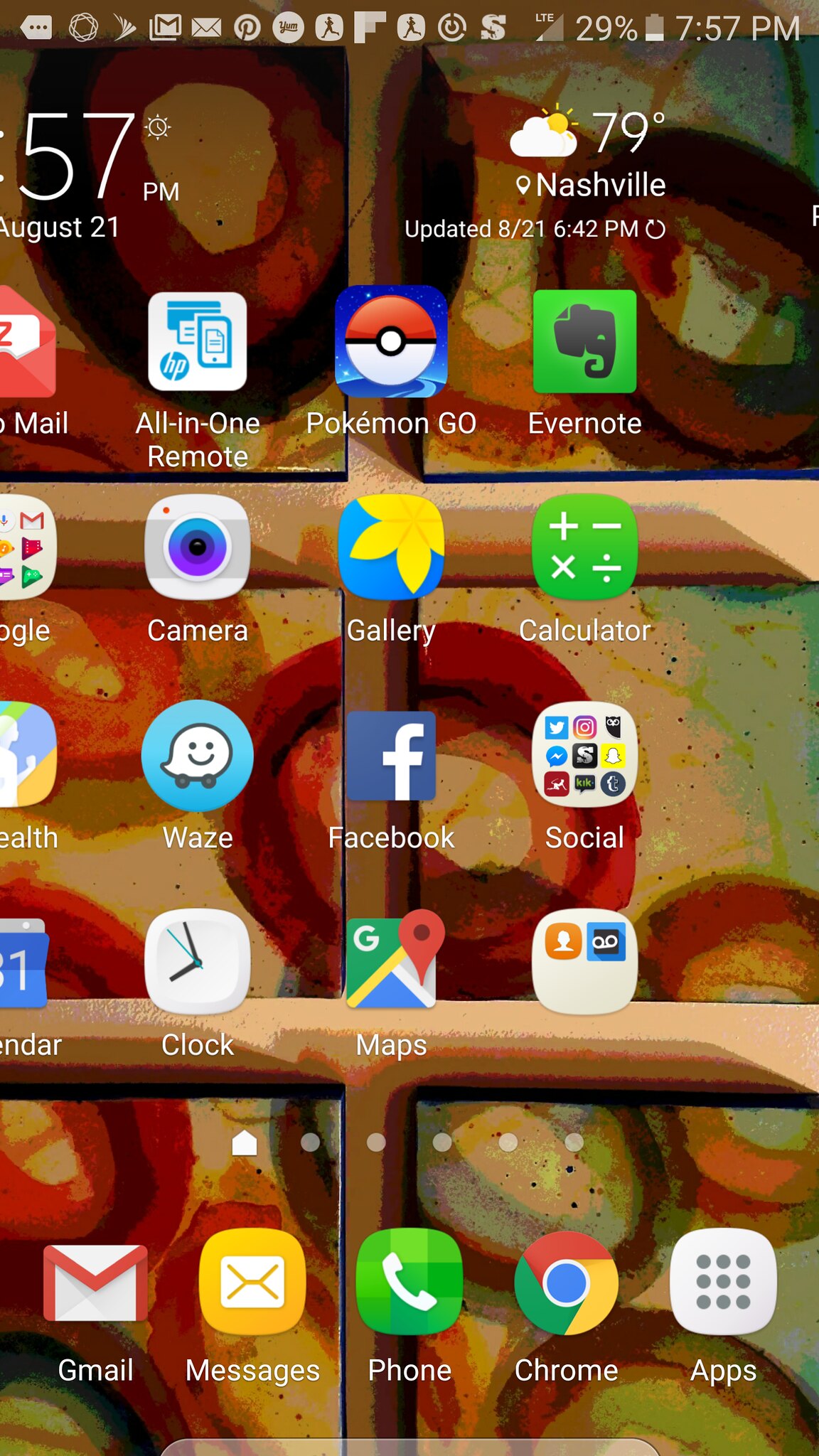This screenshot captures a smartphone's home screen with various application icons on display. At the very top, the status bar shows the current time, battery percentage, and several notification icons, all in gray text. Below this, the main section of the screen features a grid of application icons, each displaying its respective logo. The background showcases an artistic wallpaper composed of circular shapes in shades of orange, tan, and red, giving it a painted, abstract appearance. Towards the bottom, a dock contains essential applications such as the Phone app, Messaging, the Apps drawer, Chrome browser, and Gmail, indicating these are likely the user's commonly used apps.